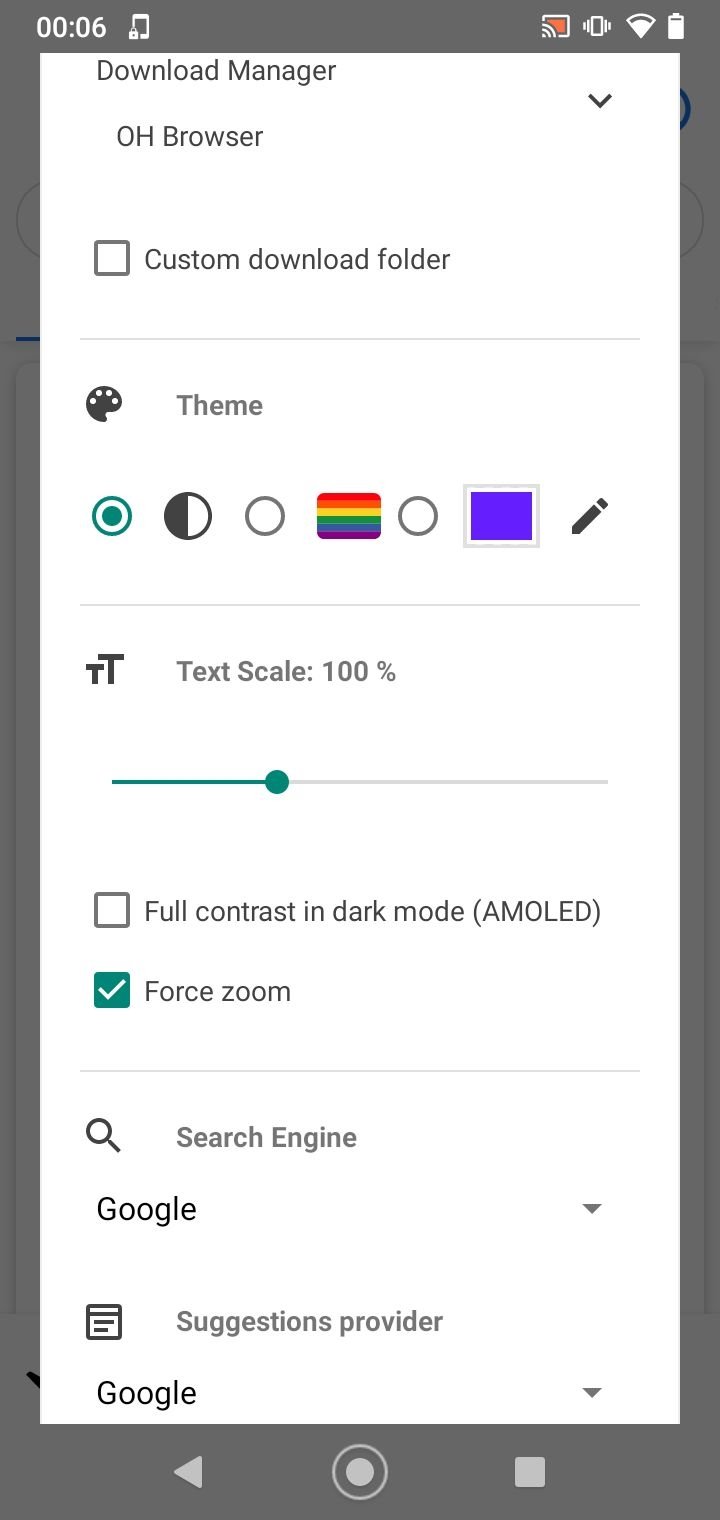The screenshot appears to be from a mobile device displaying the settings page of a download manager within the OH Browser app. The image is framed by a grey border, with a status bar at the top displaying various icons and indicators. On the left corner, the time reads "0:06," accompanied by an indistinct phone icon. Moving right, there is a red square icon likely indicating vibrate mode, followed by the Wi-Fi symbol and a nearly full battery icon.

The bottom of the screen shows navigation buttons: a back arrow enclosed within a circle and an adjacent square button, both set against a whitish-grey background.

Dominating the screen is a white background with black text. At the top, the header reads "Download Manager" with a downward arrow next to it, accompanied by "OH Browser." Below, an unticked checkbox is labeled "Custom Download Folder." Between sections, thin horizontal lines separate the different settings options.

The "Theme" section features a black and white theme icon on the left. The first theme, represented by a black and white circle, is selected. The other two themes, symbolized by a rainbow-colored rectangle and a purple rectangle respectively, remain unselected. An edit icon in the form of a pencil sits next to this section.

Further down, under another thin horizontal line, a text icon shows two "T"s of differing sizes, denoting "Text Scale" set to 100% with a slider positioned about one-third to the right. The slider itself is green on the left side with a green button, transitioning to grey on the right.

Additional settings include an unchecked checkbox for "Full Contrast and Dark Mode, AMOLED," alongside a green-ticked checkbox for "Forced Zoom." Another horizontal line leads to the "Search Engine" field, displaying Google as the selected option from a drop-down menu. The "Suggestions Provider" section beneath it also shows Google as the selected option, marked by a small square icon to its left.